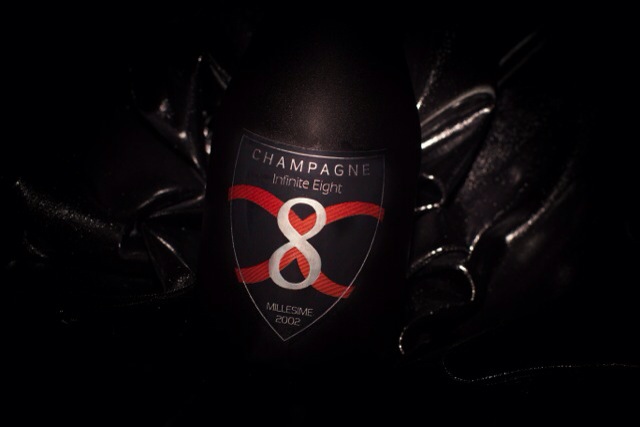This is a detailed photograph of a bottle of Champagne Infinite 8, captured in an indoor setting with a dark and sophisticated atmosphere. The champagne is presented in an opaque black bottle, exuding elegance and luxury. The label on the bottle features striking silver lettering, prominently displaying the words "Champagne Infinite 8 Millésime 2002." The label's design includes a large number 8, intersected by four crisscrosses, rendered in white and contrasting sharply against the black background. Additionally, intricate silver accents and other silver handwriting embellish the label, enhancing its refined appearance. The bottle is set against a piece of black material with white lines running through it, seamlessly blending into the solid black background and amplifying the visual impact of the composition. Highlights of red and gold on the label and possibly gold accents or ribbons on the sides further underscore the opulence of the presentation. The image, while dark and moody, effectively showcases the luxurious and classy aura of the Infinite 8 Champagne.